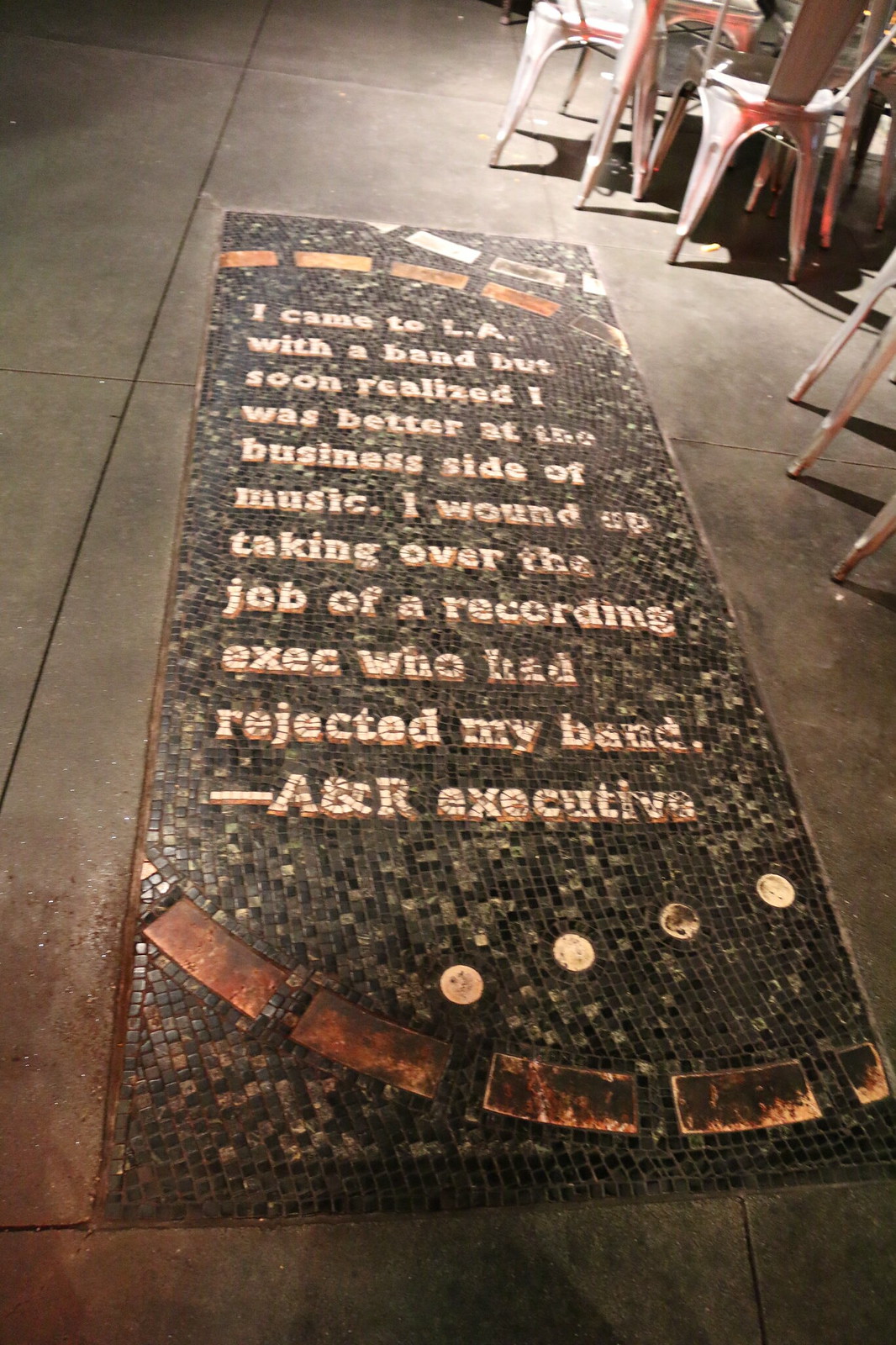This nocturnal city street scene captures an atmospheric urban setting bathed in the soft glow of streetlights against a darkened sky. To the right, white metal chairs and tables suggest a casual outdoor dining area, adding to the street's lived-in charm. The foreground and left remain clear, drawing attention to a compelling centerpiece on the gray-black sidewalk. An artistic mural, crafted from tiles and various other materials, dominates the middle of the scene. Inscribed within the mosaic tiles is a poignant message: "I came to LA, meaning Los Angeles, with a band but soon realized I was better at the business side of music. I wound up taking over the job of a recording exec, meaning executive, who had rejected my band." This reflective and personal statement is attributed to an A&R Executive, offering a narrative of transformation and resilience embedded within the urban artwork.